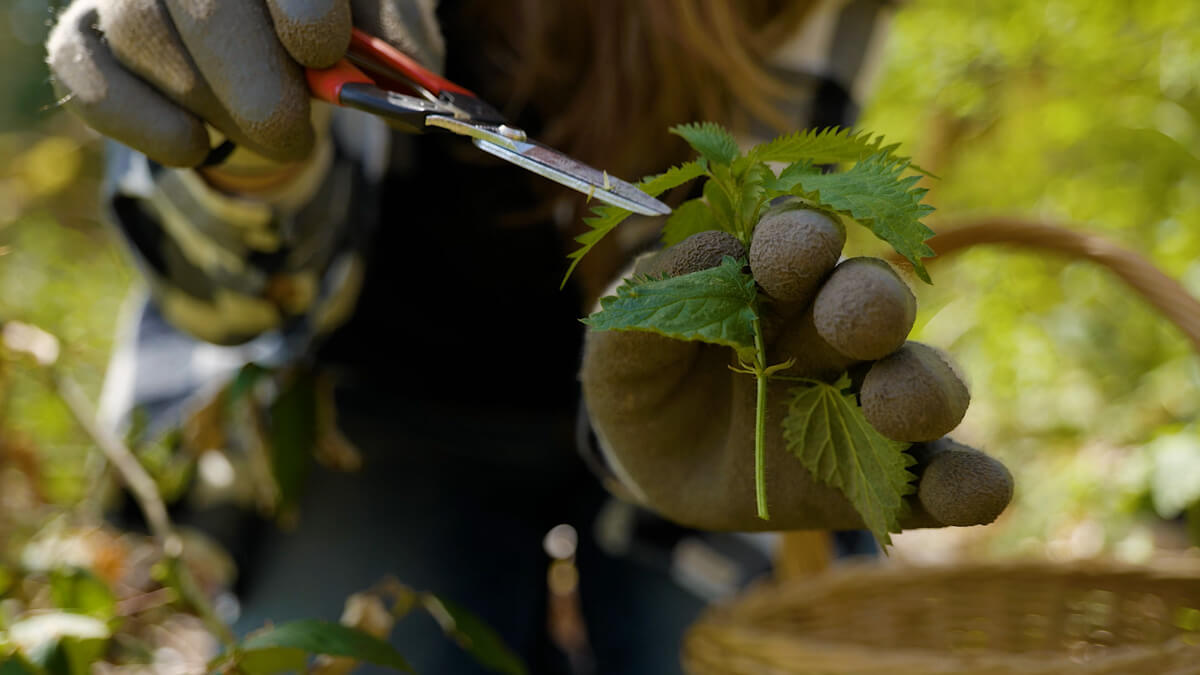In this detailed photograph, a gardener, likely a female, works diligently amidst a lush, green area, which might be a forest. She is wearing dark gray or olive-colored gloves and wielding a pair of silver-bladed scissors to carefully cut the tips or leaves of vibrant green plants. Her long hair suggests her gender, although her face remains out of sight as the camera focuses intently on her meticulous work. A light beige woven basket is positioned beside her, hinting that she is collecting and possibly sorting these plant pieces, perhaps removing any unwanted or poisonous sections. The blurred greenery in the background emphasizes the natural setting, underscoring her careful, methodical approach to handling the plants.